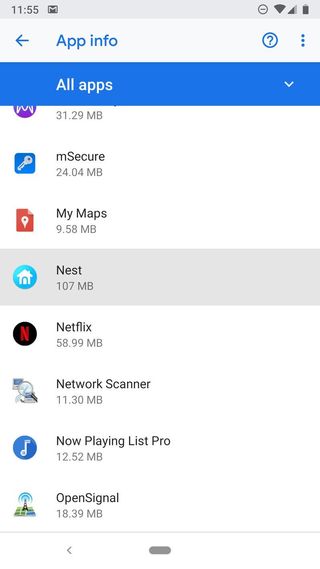A detailed screenshot of a smartphone’s app management page. The device shows the standard status bar information including the time at 11:55 AM, a new email notification, Wi-Fi signal strength, mobile network bars, and the battery level on the top right. Below, there's a header titled “App Info,” flanked by a back arrow on the left and a help icon along with a three-dot menu on the right. A prominent blue banner below the header displays “All Apps” alongside a clickable down arrow for further options.

The list of apps begins with several partially visible entries. The first app is partially off-screen but features a purple and white logo and occupies 31.25 MB of storage. Next, “M Secure” is listed with a key logo, consuming 24.04 MB. Following that is “My Maps,” identified by a map pinpoint logo, using 9.58 MB. The app “Nest,” marked with a house logo, takes up 107 MB and is highlighted with a gray background, indicating it is currently selected. “Netflix,” sporting the recognizable Netflix logo, is using a substantial 5899 MB. Below this is “Network Scanner,” which has a detailed logo, potentially featuring a computer and magnifying glass, at 11.30 MB. “NowPlayingList Pro” appears next, associated with a music icon, taking up 12.52 MB. Lastly, “OpenSignal,” marked by a Wi-Fi or radio tower icon, uses 18.39 MB of storage. At the bottom of the screen, a back button is partially visible, suggesting navigation options to return to the previous menu.